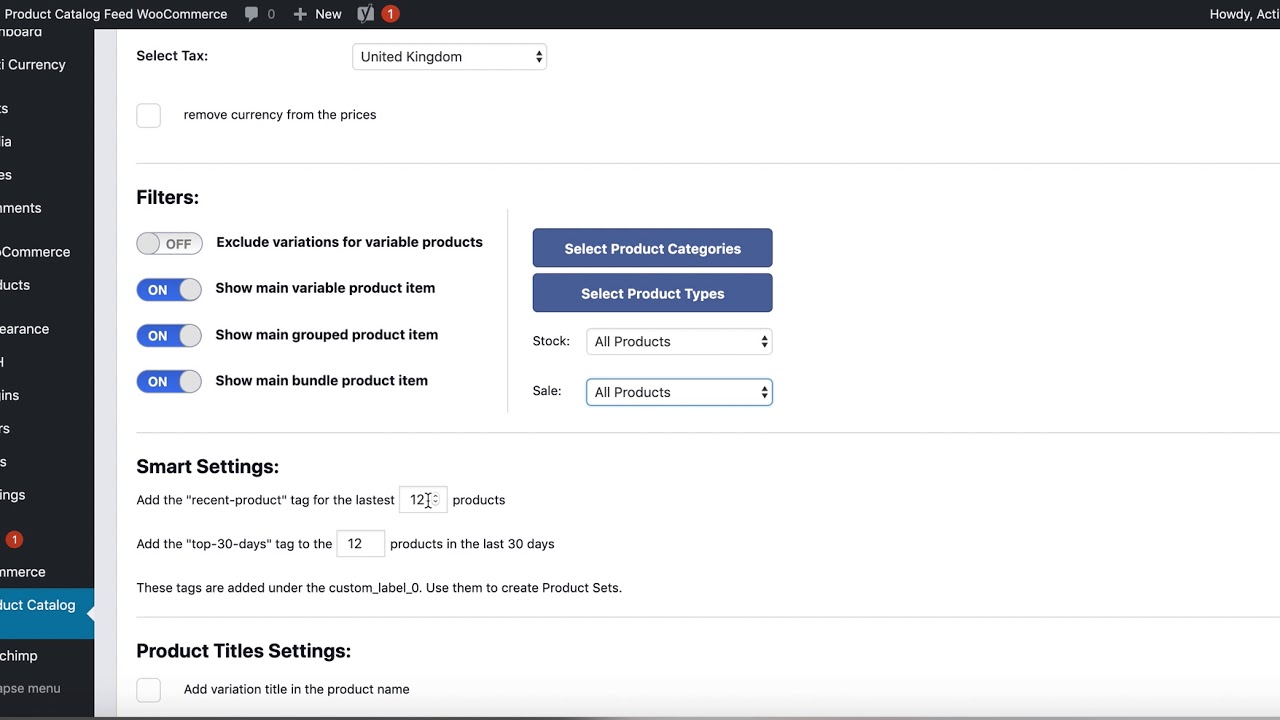This image is a screenshot displaying a partially visible navigation bar on the left side, which includes partially readable menu items like "Dashboard," "Currency," "Commerce," "Catalog," and "Menu." The top section features a black border with text and icons including "Product Catalog Feed," "WooCommerce," a message icon, and a notification badge displaying the number 1 in a red circle. The main content area, set against a white background, showcases various interface elements and settings. On the left, there are filters with toggle switches, all switched on, labeled "Show Main Variable Product Item," "Show Main Grouped Product Item," and "Show Main Bundle Product Item." Adjacent to these toggles are two action boxes labeled "Select Product Categories" and "Select Product Types." This setup appears to be part of a product management or e-commerce dashboard, likely associated with WooCommerce.